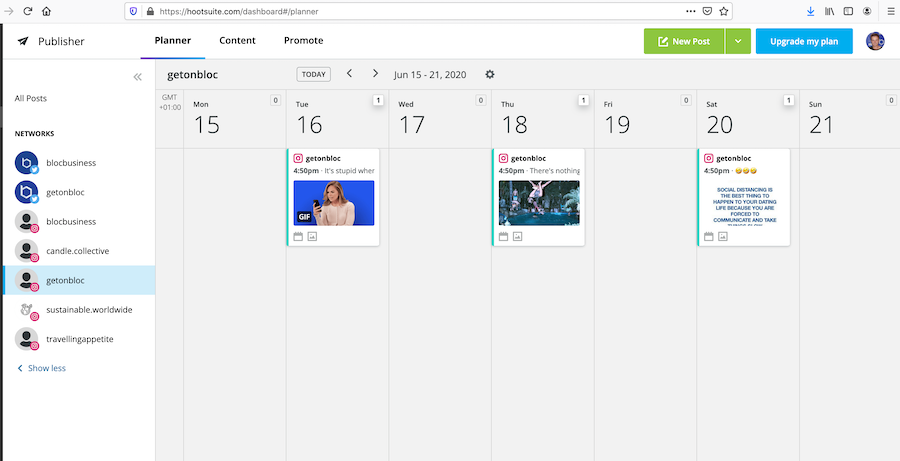The image is a detailed screen capture of a desktop computer displaying a web page from Hootsuite's Planner, accessible via the URL https://hootsuite.com/dashboard/planner. In the upper-left corner, the name of the app, "Publisher," is prominently displayed. The left window pane lists approximately seven different networks, each accompanied by profile icons and network names. The first network in the list is labeled "Block Business." 

On the right side of the window, the main section features an off-white background showcasing a calendar. The visible dates range from Monday the 15th through Sunday the 21st. Within the calendar columns for Tuesday the 16th, Thursday the 18th, and Saturday the 20th, there are entries indicating scheduled activities or posts.